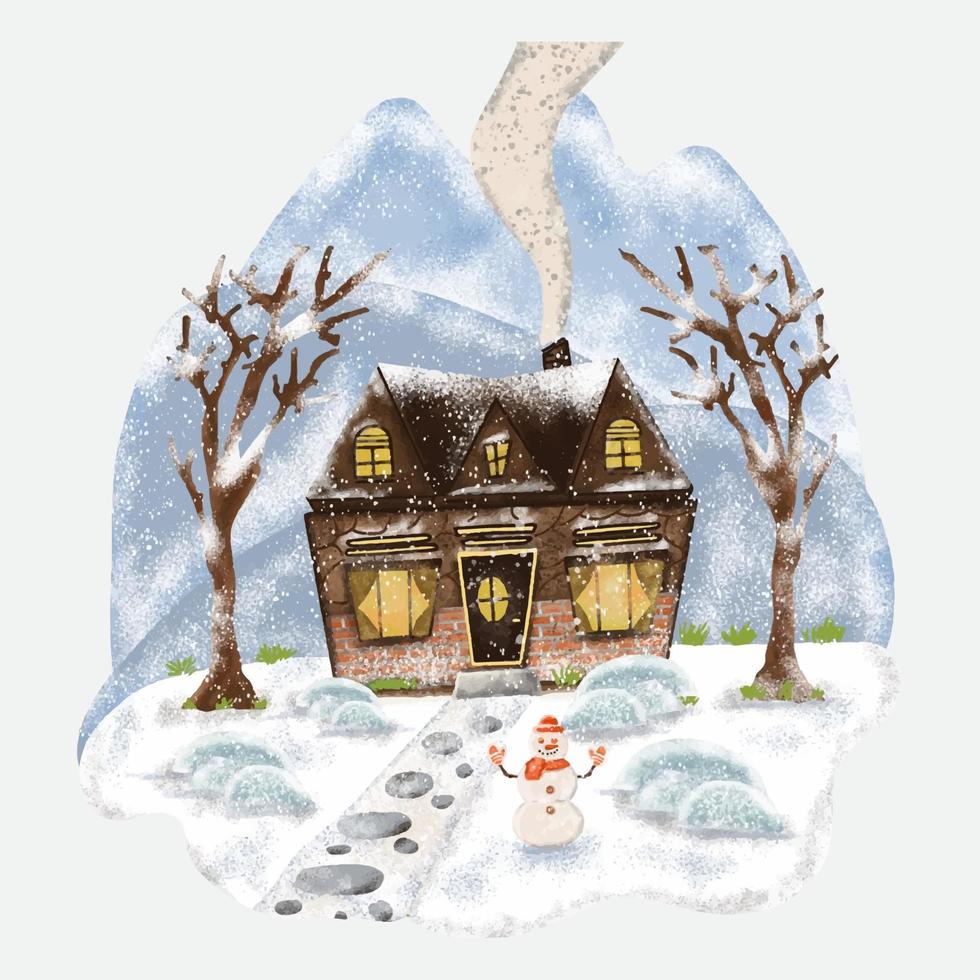This digital illustration vividly depicts a charming winter scene on a blue-gray snowy backdrop, resembling something fit for a Christmas card. At the heart of the image stands a cozy two-story house, characterized by its brown façade and red brick lower half. The house features six warmly lit windows, casting a yellow glow, and a door with a unique trapezoidal shape, topped by an oval glass pane. A plume of smoke curls skyward from the chimney, adding to the homey atmosphere.

Flanking the house are two bare trees, their brown branches stark against the snowy expanse. In the foreground, a cobblestone pathway, made up of round pavers, winds through a blanket of snow towards the house. This pathway is bordered by mounds of snow-covered shrubbery, suggesting evergreen bushes underneath.

In the front yard stands an endearing snowman, complete with a traditional carrot nose, coal eyes, and a delighted rock smile. The snowman is adorned with a red cap, matching red scarf, and red mittens on its twig arms. Snowflakes gently fall throughout the scene, contributing to the serene winter wonderland ambience. The background is subtly detailed with hints of snow-capped hills or mountains, adding depth to this picturesque winter tableau.